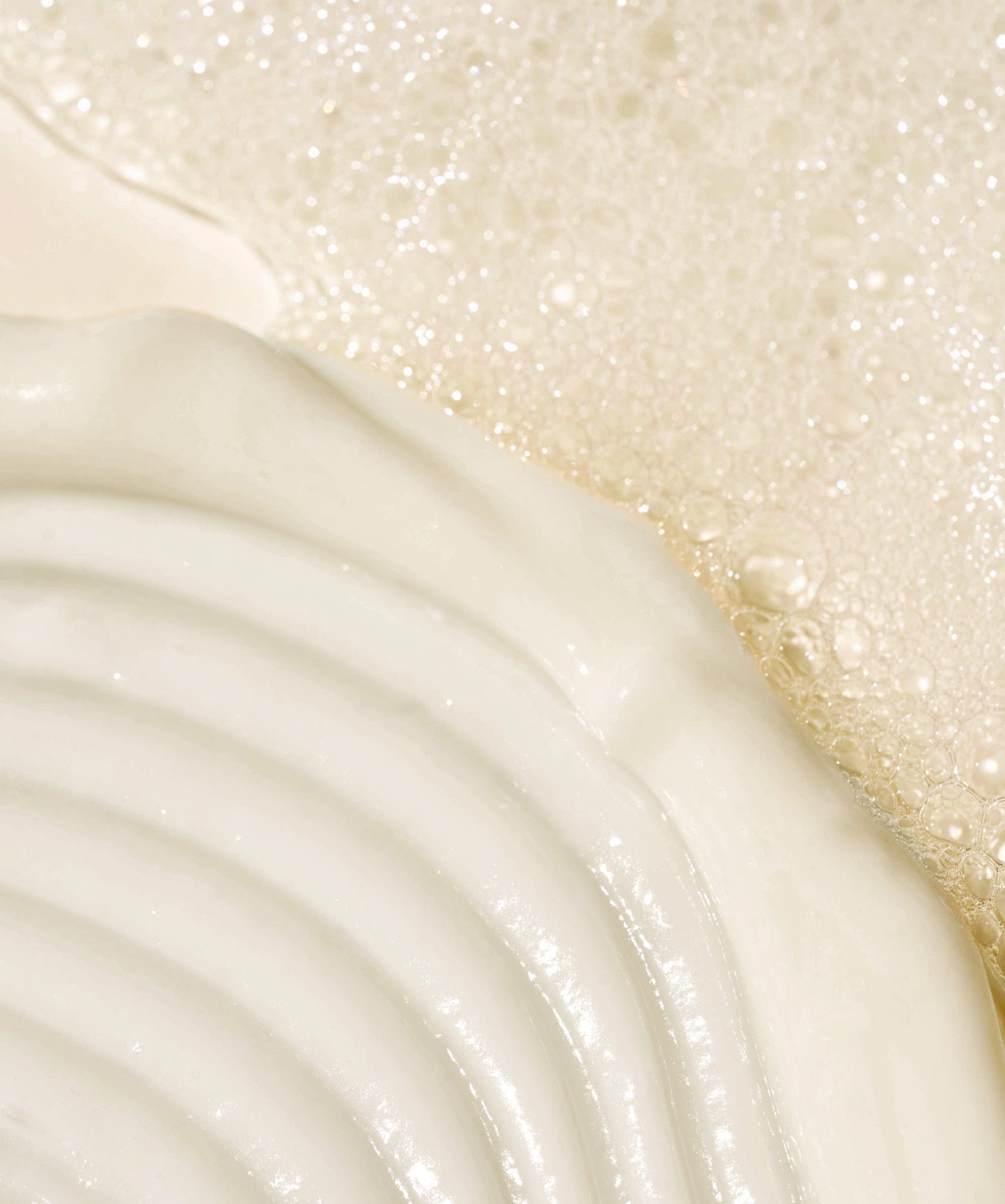This rectangular, borderless image is a detailed close-up photograph of a bubbly and creamy substance, likely some kind of soap or lotion. The lower left of the image features swirls of a beige-colored cream, showing intricate textures that resemble a combed pattern. The upper right area of the photo is filled with hundreds, possibly thousands, of clear and white bubbles with brown edges, giving the surface a crystally appearance. These bubbles form a textured, solid-looking triangle that extends back up towards the upper left side. The thickest part of the material stretches diagonally from the upper left to the lower right. There is no text in the image, and the lighting appears to be coming from behind the camera, casting soft highlights on the substances.